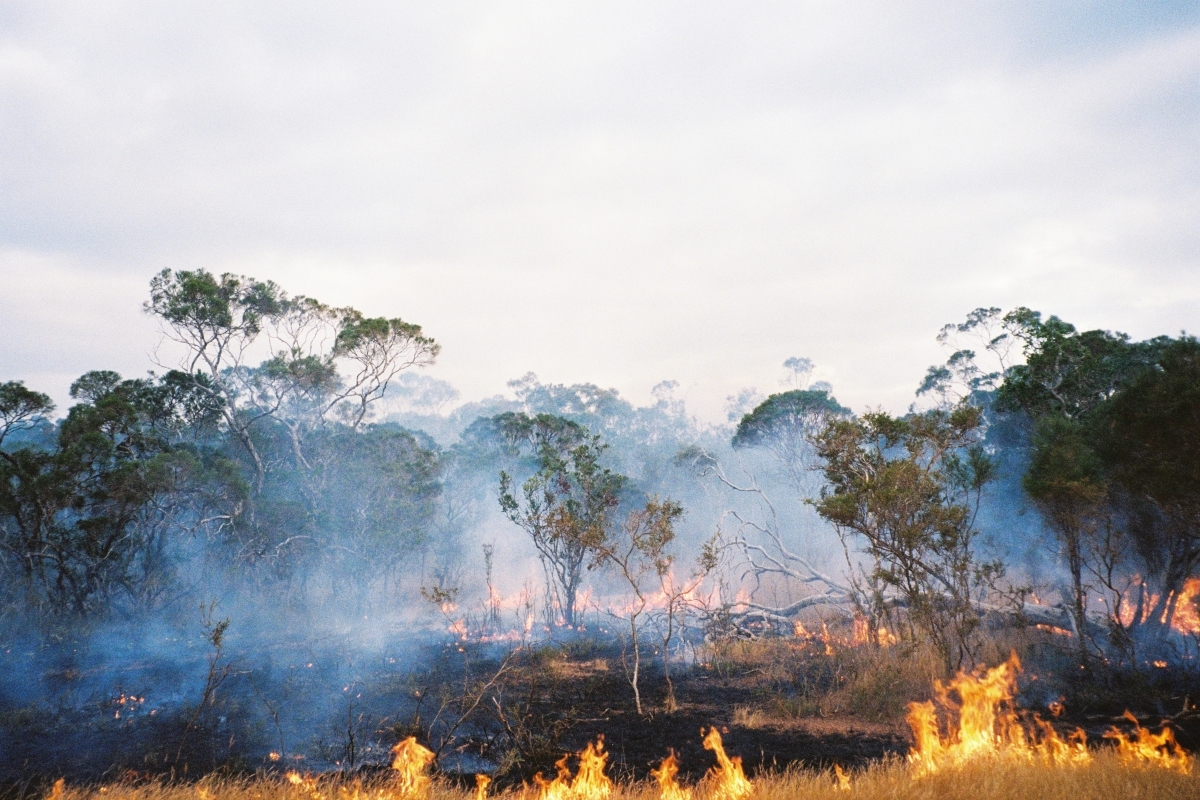The photo depicts a devastating forest fire, likely occurring in the Amazon or a similar rainforest. The top half of the image is dominated by a smoky, cloudy sky, the smoke rising thickly into the atmosphere and obscuring much of the natural light. Moving towards the bottom, the scene transitions to a mix of burning trees and ignited grassy plains, with flames licking up from the underbrush. The central portion of the image reveals the heart of the destruction—numerous trees at varying stages of combustion, shrouded in dense smoke that masks parts of the background. Charred remnants and hot coals are scattered throughout, indicating that the fire, while still active, might be in its later stages with flames less rampant than before. The overall atmosphere is one of bleak devastation, with the once-vibrant forest now a smoldering and smoky battlefield.